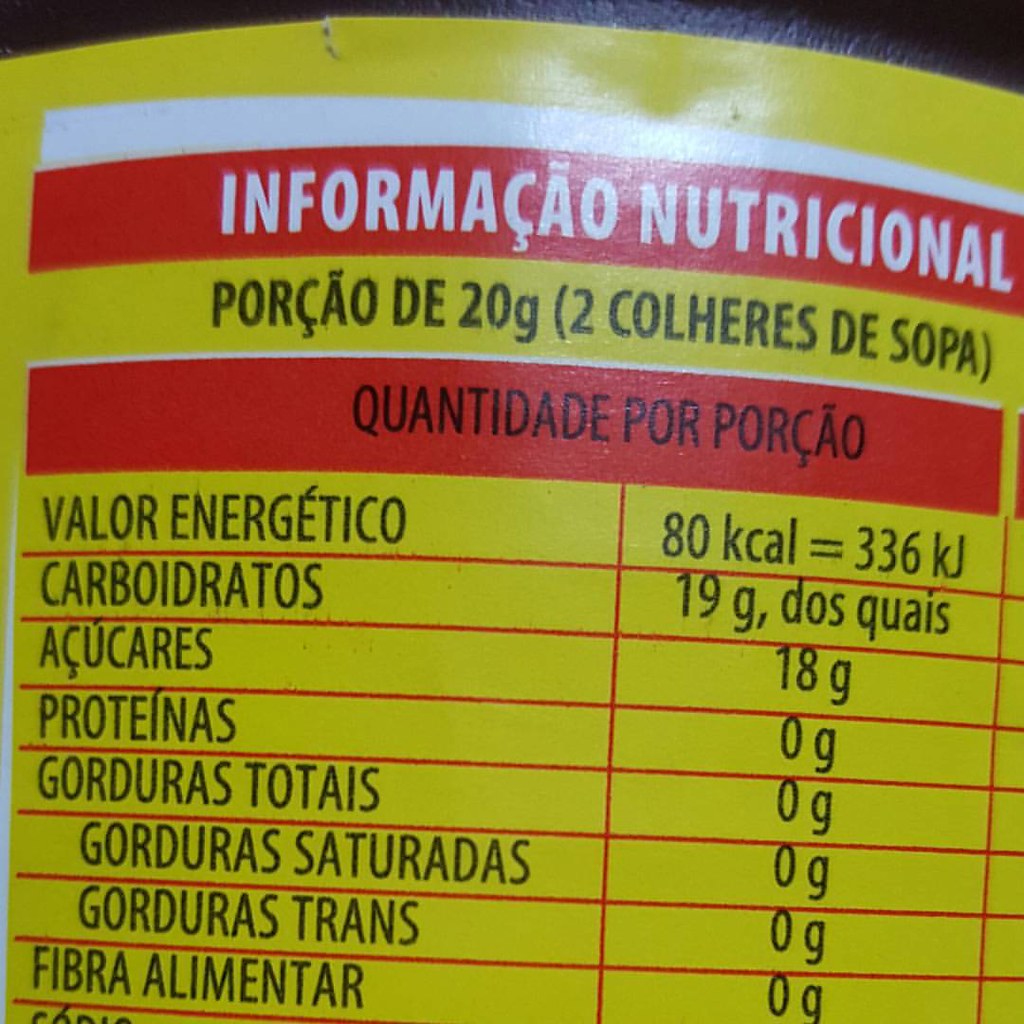The image depicts a detailed nutritional information label predominantly featuring a bright yellow background, framed by a series of horizontal stripes. The top portion of the label has a slight white border, followed by a prominent red strip with white text that reads "Información Nutricional," indicating that the nutritional data is in Spanish. Below this red strip, the label contains a yellow section that lists the nutritional components, each separated by fine red grid lines. The left column lists various nutritional elements, such as calories, carbohydrates, and proteins, with their corresponding amounts on the right side, displaying measurements like 80 kcal (equivalent to 336 kJ), 19 grams, and 0 grams for certain nutrients. There is another red section towards the bottom of the yellow portion, continuing the informational details. The label appears to be adhered to a dark-colored surface, with a small rip visible at the top left corner of the label. The vibrant and organized layout makes the nutritional facts easily readable, despite being in a foreign language.